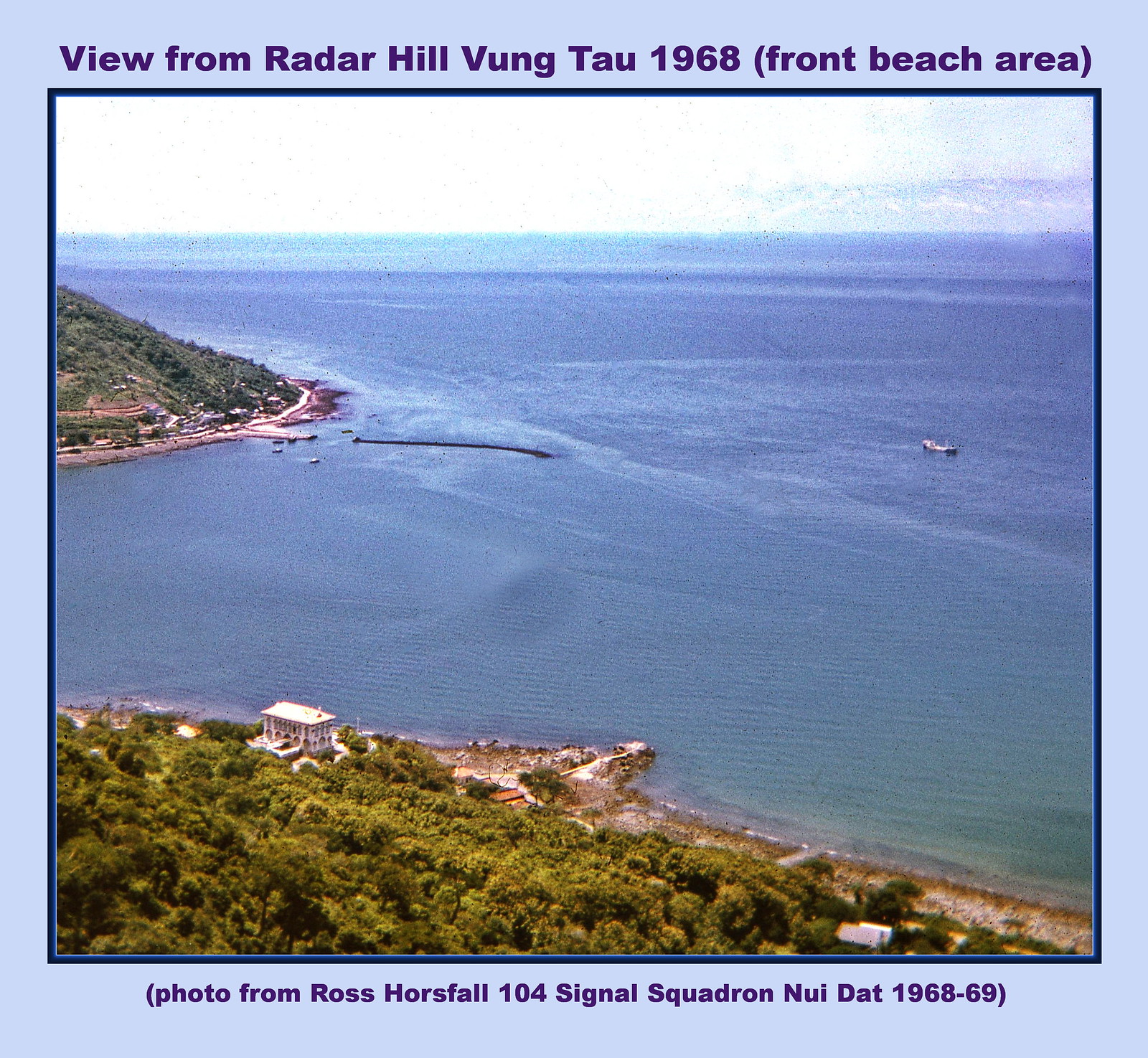This vintage photograph, framed in dark blue, captures a panoramic view from Radar Hill, Vung Tau, 1968, during the Vietnam era, with annotations in purple stating it is a "view from Radar Hill, Vung Tau, 1968 (front beach area)" and crediting "photo from Ross Horse Fall 104 Signal Squadron, 1968-69." The image, slightly yellowed and faded, appears to be taken from a high vantage point, possibly a helicopter. It depicts a picturesque bay area with the ocean extending inland, creating a harbor-like inlet. 

In the top left corner, land juts out into the water, its dense covering of trees giving way to some nearby structures along the beach level. A large manor, presumably white with possible columns, stands prominently on the shoreline amidst other smaller buildings. The beach transitions to rocky terrain along the water’s edge, where a jetty with a walkway extends outward. A wall-like structure in the water suggests a harbor area. Multiple boats dot the ocean, especially in a bustling section at the top of the image, indicative of a crowded pier area. The overall scene portrays a lush, tree-lined hill on the left and broad, blue ocean waters varying in shades, emphasizing the historical and serene atmosphere of the Front Beach area in Vung Tau.